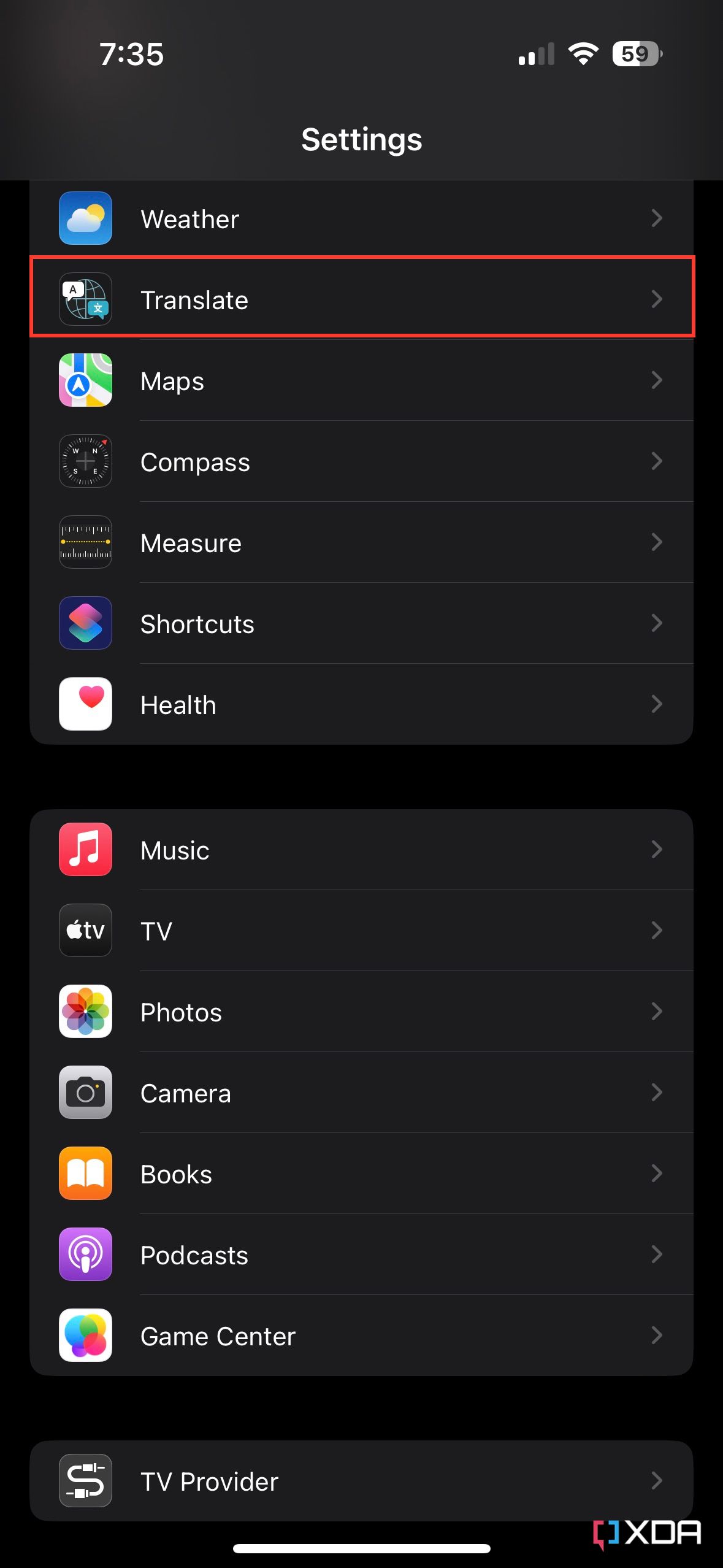The image displays the settings menu on a cell phone with a timestamp at the top indicating it is 7:35. The background is black, and the word "Settings" is prominently displayed in white letters at the top.

Below the main heading, a list of various apps is shown:

1. **Weather**: Features a blue background with a yellow sun and a white cloud icon.
2. **Translate**: Highlighted with a red border.
3. **Maps**: Displays the standard maps icon.
4. **Compass**: Includes a compass icon.
5. **Measure**: Represented by a tape measure icon.
6. **Shortcuts**: Shows the shortcuts icon.
7. **Health**: Contains a pink heart on a white card.
8. **Music**: Depicts the Apple Music logo with a red background and a white music note.
9. **Apple TV**: Features the Apple TV icon, an Apple symbol alongside "TV."
10. **Photos**: Shows the Apple Photos icon.
11. **Camera**: Displays the Apple Camera icon.
12. **Books**: Depicted by an orange icon with a white book.
13. **Podcasts**: Features a purple square with a white podcast logo.
14. **Game Center**: Displays the Game Center logo.
15. **TV Provider**: Has a cord icon.

Each app icon is clearly displayed against the dark background, making them easily identifiable.